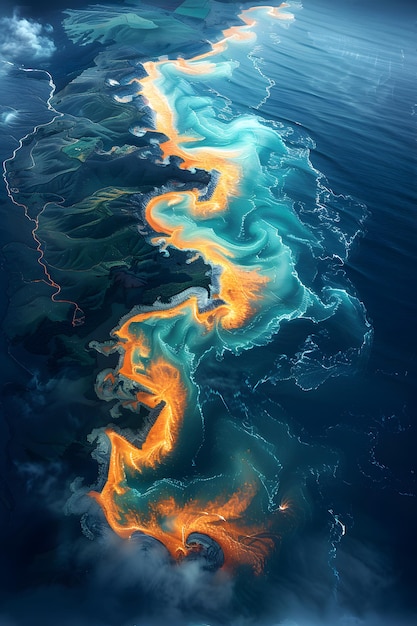The image features a digitally enhanced aerial view of a dramatic island landscape. The island's geography includes a mountainous western side covered with lush, green terrain, contrasting starkly with the east side, which is dominated by a fiery lava flow. The lava, rendered in rich orange tones, cascades from north to south, creating a striking golden stream that meets the ocean. As the molten rock touches the water, it generates a spectacle of greenish, foamy wave patterns. The eastern shoreline is characterized by bays and peninsulas tinged with fiery orange streaks, giving the appearance of a volatile, eruptive landscape. Above, misty white clouds drift, adding a surreal layer to the panoramic view, which combines elements of both a photograph and intricate graphic design. The predominant colors in the scene are darkish blue, turquoise, and orange, creating a vivid depiction of nature's contrasting elements.